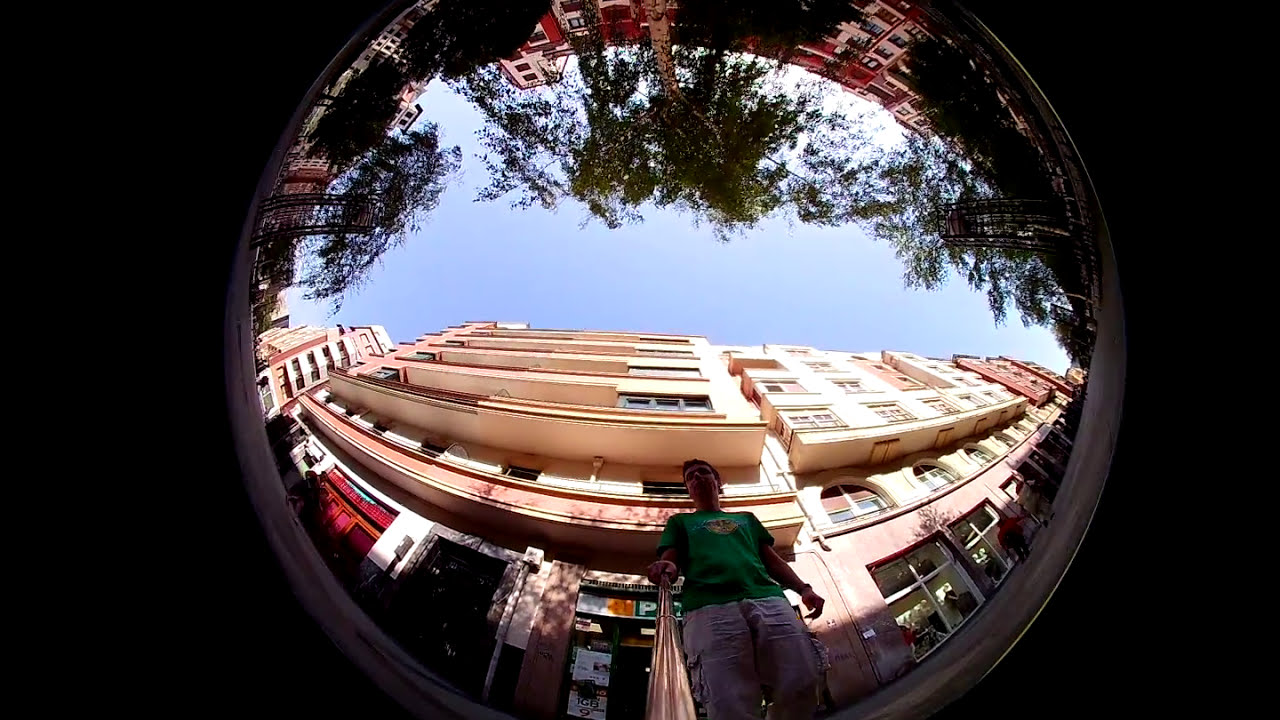The photograph appears to be taken from a unique perspective, as if the camera is positioned inside a circular manhole or pothole on the ground, looking upward. The surrounding edges of the image are black, giving the impression of peering through a tunnel. A man, wearing a green t-shirt, possibly featuring a logo, and khaki shorts or pants, stands above the camera, looking down at it. He is holding what seems to be a silver selfie stick or a gold pole. Surrounding him are various tall buildings with storefronts at the bottom, large windows, balconies, and signage, suggesting they house both commercial and residential spaces. The buildings exhibit colors like red, brown, and white. In the background, the sky is clear and bright blue, with a few clouds and the tops of green-leaved trees visible. Other details include people in the background, walking on a gray sidewalk, and a mix of signage including a letter 'P' on a green background.